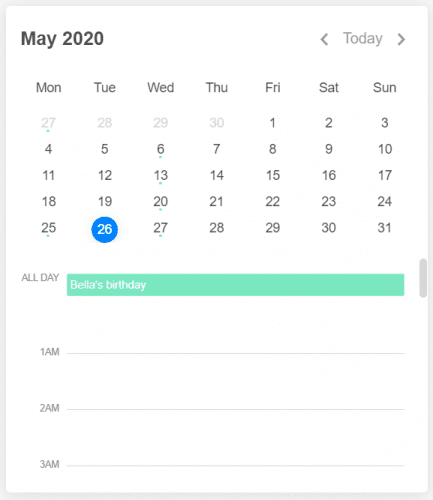In the top left corner, the date "May 2020" is displayed in black text. Moving to the right, there is a small arrow pointing left, followed by the word "Today" and another small arrow pointing right. The days of the week are abbreviated and listed horizontally: MON for Monday, TUE for Tuesday, WED for Wednesday, THU for Thursday, FRI for Friday, SAT for Saturday, and SUN for Sunday. 

The date highlighted is Tuesday the 26th, found in the last row of dates. The number 26 is inside a blue circle, with the digits in white. Below this, it is indicated that the event lasts "All Day." To the right is a long, greenish-blue rectangle with the text "Bella's Birthday" inside. 

Further down, the times 1 a.m., 2 a.m., and 3 a.m. are listed sequentially, each accompanied by a long gray line. The calendar's provided information ends at 3 a.m.